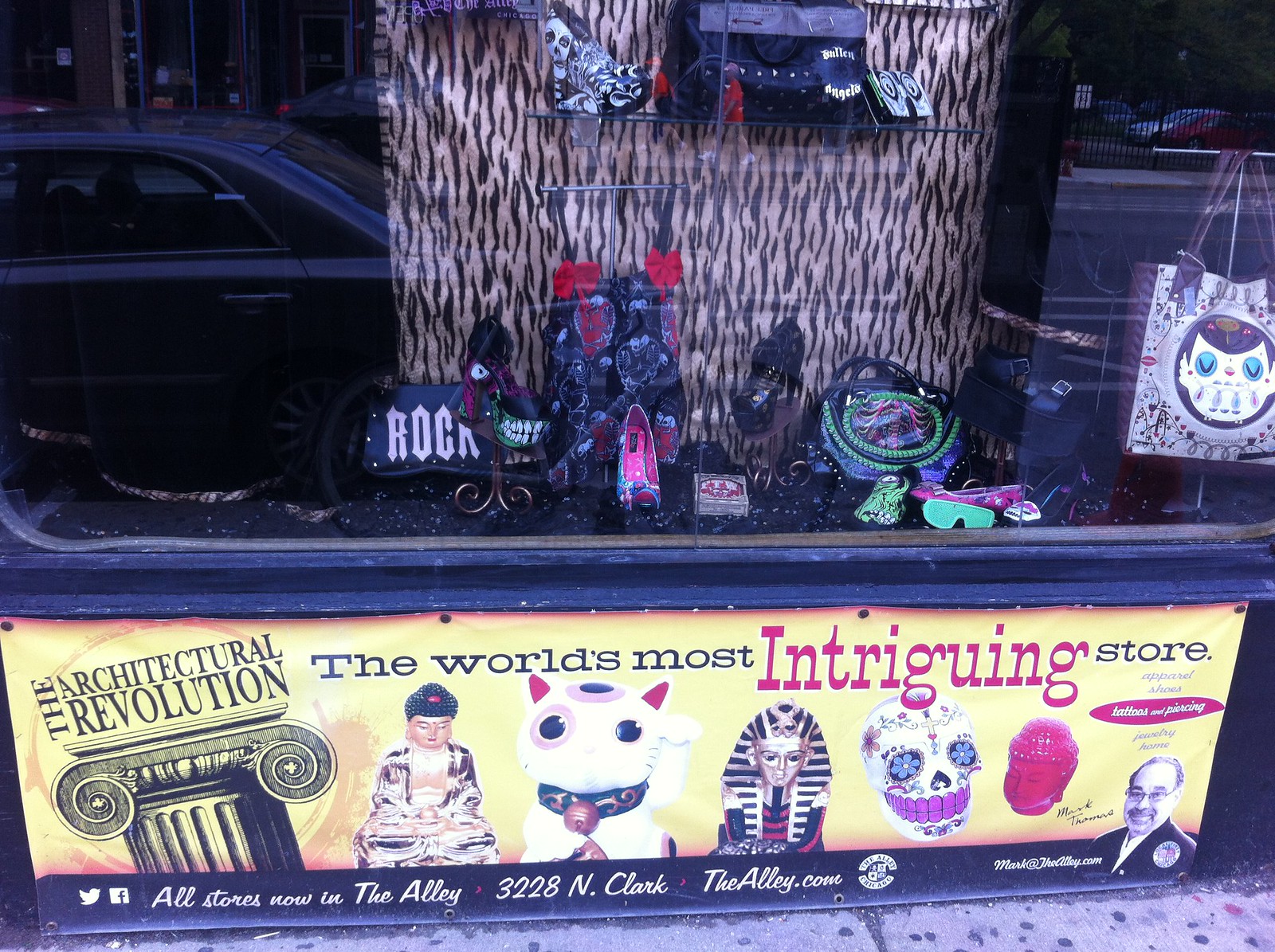The image depicts a storefront display on a city street, viewed through a reflective glass window. The reflection includes parked cars and buildings. Inside the display, prominent elements include a pair of high heel shoes, vibrant handbags, and various accessories featuring bold, multi-colored designs. The background of the display showcases a light purple curtain with white vertical streaks.

On the left side of the display, a handbag with green and blue circular patterns is visible, adjacent to a hanging shopping bag adorned with a face illustration and marked by a purple color scheme. Beneath the display, a banner with a yellow background reads, "The Architectural Revolution," accompanied by an illustration of a Roman column. Above this, the text "The World's Most Intriguing Store" is featured prominently in bold purple font.

The banner further includes images of eclectic products such as a Buddha statue, a waving cat statue, a Pharaoh bust, a skeleton with big blue eyes, and a red Buddha head. In the bottom right corner, a black and white photo of a man, the proprietor, is displayed. The bottom of this banner has a black border listing social media icons, location details (including 3228 North Clark and thealley.com), and the store's email address.